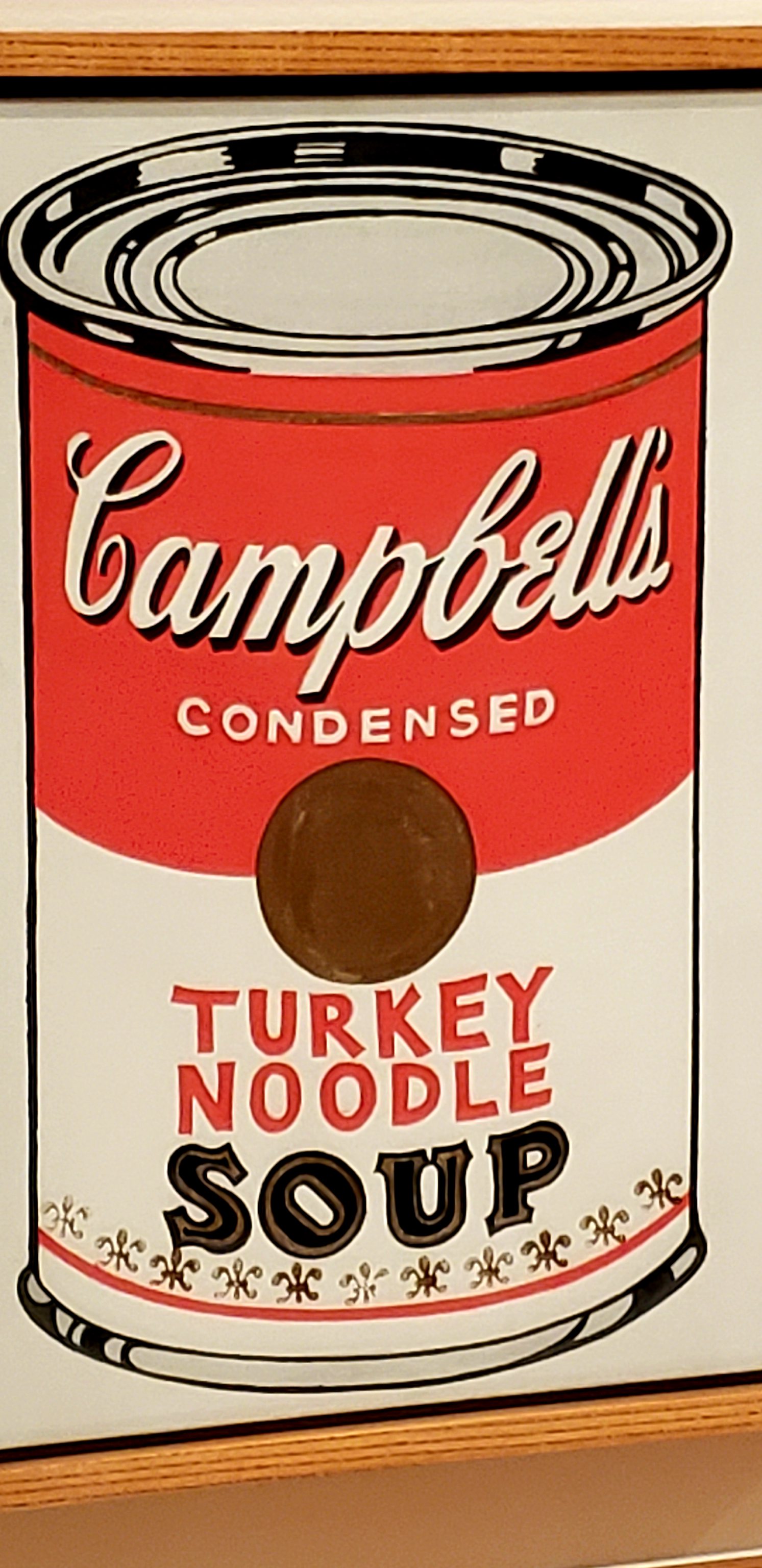This illustration features a Campbell's Condensed Turkey Noodle Soup can, rendered in a stretched portrait orientation. The Campbell's brand name is prominently displayed at the top in its iconic script. The upper half of the can is a bright red, accentuated by the white text "Campbell's Condensed," with a small brown dot separating the words "Condensed" and "Turkey." Below, the label transitions to a white background that hosts the product's name "Turkey Noodle" in red letters and the word "Soup" in bold black letters. Adding a touch of charm, a decorative row of small flowers is situated just beneath the word "Soup," completing the classic and recognizable design of this Campbell's product.